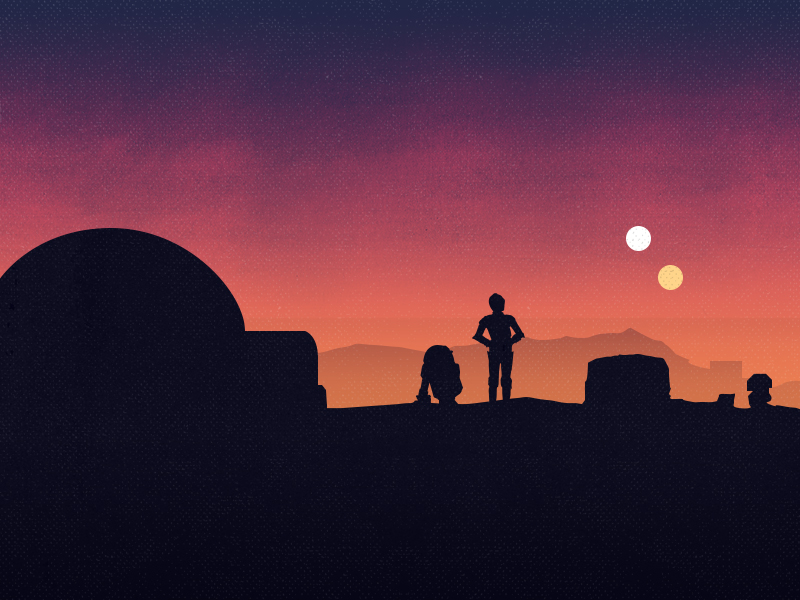This image, which appears to be a still from a Star Wars movie, depicts the iconic droids C-3PO and R2-D2 silhouetted against a stunning sunset. The pair stand on the rooftop of a rounded structure, reminiscent of an astronomy observatory. The skyline features two celestial bodies, one brighter than the other—likely Tatooine's twin suns. The sky transitions through a vivid ombre of dark navy blue, purple, pink, and salmon hues, casting a hazy, almost surreal light over the scene. In the distance, a range of mountains and hills adds depth to the composition, while the overall atmosphere captures a moment of contemplation as the droids gaze out over the serene, extraterrestrial landscape.